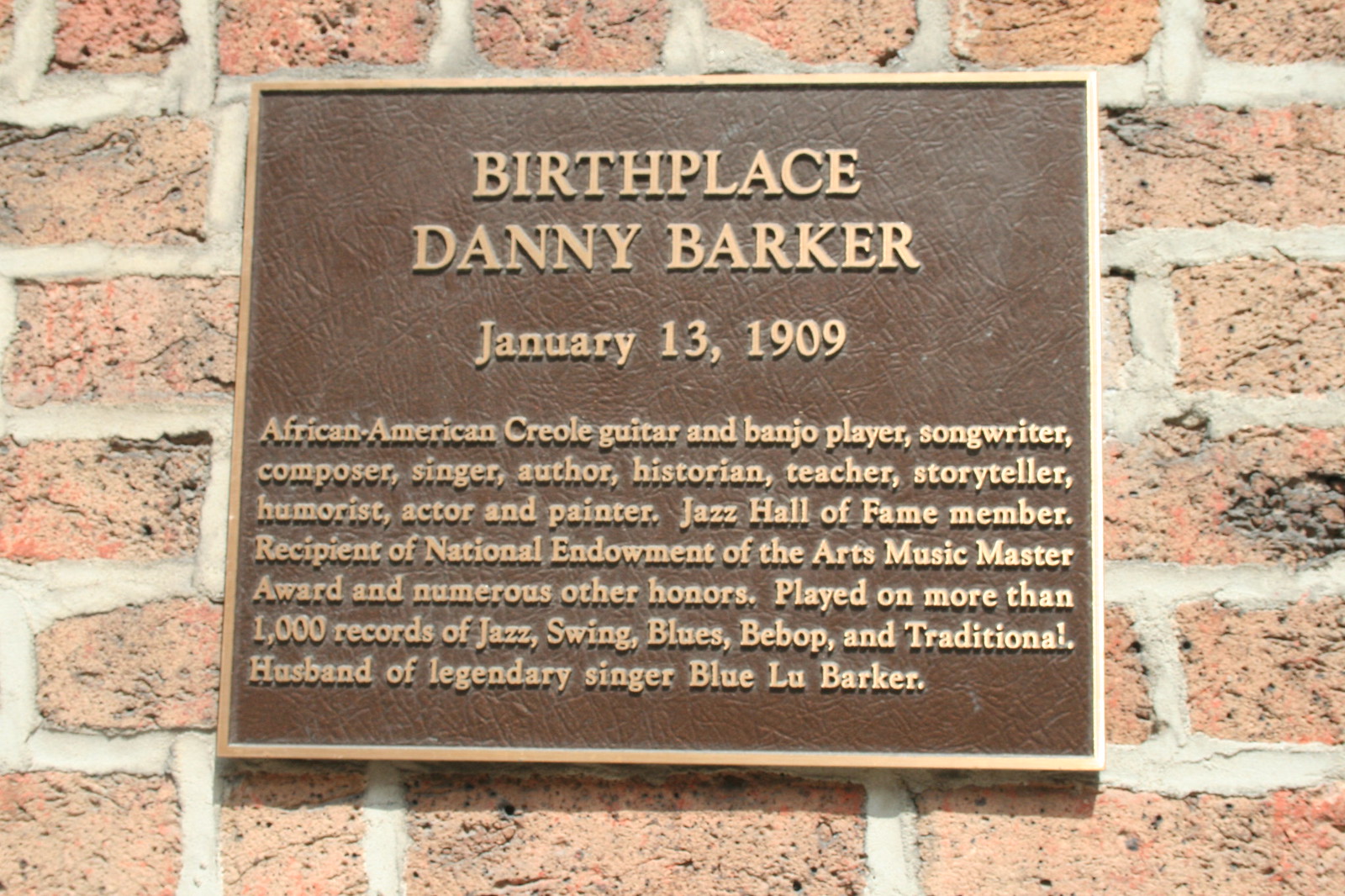The image features a square bronze-outlined plaque mounted against a brick wall. The plaque, with a brown interior, prominently displays text that reads: "Birthplace of Danny Barker, January 13th, 1909." Below this, smaller text honors Danny Barker as an African-American Creole guitar and banjo player, songwriter, composer, singer, author, historian, teacher, storyteller, humorist, actor, and painter. It highlights his achievements as a Jazz Hall of Fame member and the recipient of the National Endowment for the Arts Music Master Award, along with numerous other honors. It also notes that he played on more than 1,000 records encompassing jazz, swing, blues, bebop, and traditional music, and acknowledges him as the husband of the legendary singer Blue Lou Barker. The plaque's elegant framing in gold further accentuates its significance.